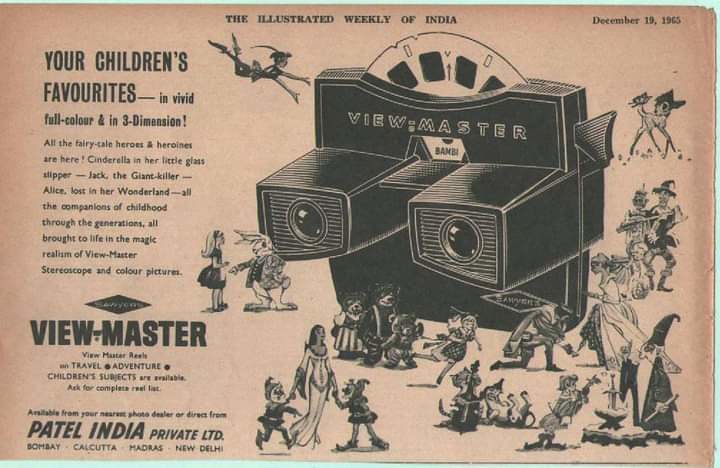A nostalgic, close-up view highlights a faded, aged advertisement for the children's toy, the Viewmaster. Once white, the paper now bears a yellowish-tan hue, with occasional tinges of pinkish orange, suggesting its age. The advertisement, inked in black with hand-drawn illustrations, is emblazoned with the masthead "The Illustrated Weekly of India" in strong black letters at the very top, dated December 19, 1965, at the upper right corner.

Dominating the center is an image of the Viewmaster toy, a plastic device resembling binoculars or a camera, designed for viewing photographic slides in vivid full color and three-dimensions. The user looks through the twin lenses and operates a handle on the right to rotate the circular disc, unveiling an array of miniature images depicted in 3D.

Around the illustration of the Viewmaster, various enchanting characters from beloved fairy tales and classic stories are brought to life – Cinderella trying on her iconic glass slipper, Jack the giant killer, Alice wandering in Wonderland, and Peter Pan soaring towards the scene. Additional illustrations feature figures such as Bambi with a butterfly on his tail, the Scarecrow and Tin Man walking together, and a young boy attempting to pull the sword from the stone.

Accompanying the visuals, the text joyfully proclaims: "Your children's favorites in vivid full color and three-dimension! All fairy tale heroes and heroines are here. Cinderella in her little glass slipper. Jack the giant killer. Alice lost in Wonderland. All companions of childhood through the generations. All brought to life in the magic realm of ViewMaster. Stereoscope and color pictures."

The bold text "Viewmaster" spans beneath this flourish, emphasizing the product’s brand. Below, a call to action reads: "ViewMaster reels with travel, adventure, children's subjects are available. Ask for complete reel list." Consumers are directed to seek these delightful reels from their nearest photo dealer or directly from Patel India Private Limited in Bombay, Calcutta, Madras, and New Delhi.